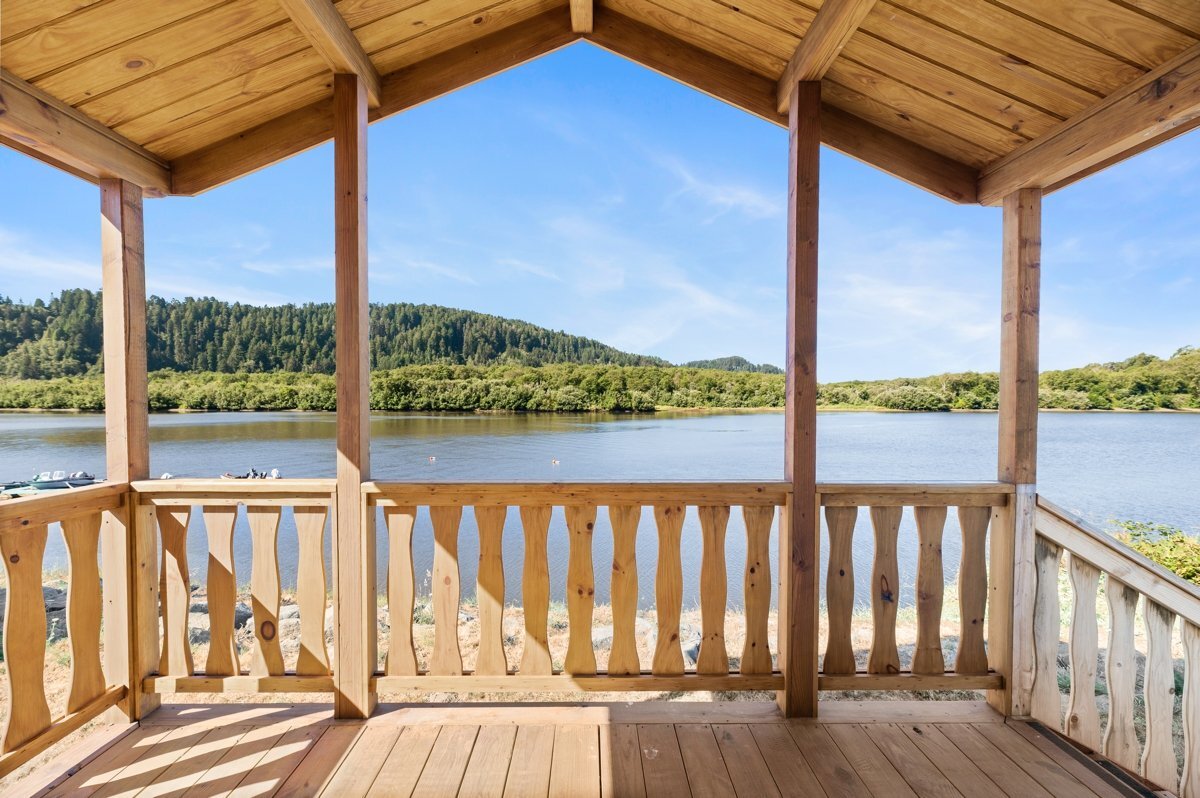This image captures a beautiful outdoor scene taken from underneath a rustic wooden gazebo or covered porch situated right on the beach of a serene lake. The structure features natural, new-looking light wood with four large beams supporting the roof and a sturdy railing. There is a staircase leading down to a sandy beach area to the right. To the left, a boat is moored while ducks and geese float peacefully on the clear blue water beneath a sky dotted with wispy clouds. The distant shoreline is lush with green shrubbery and trees that transition into gently rolling hills. A few bushes are visible near the base of the stairs, adding to the natural charm of the setting. The overall atmosphere is one of tranquility, with the inviting lake and picturesque surroundings offering a perfect spot for picnicking and relaxation.